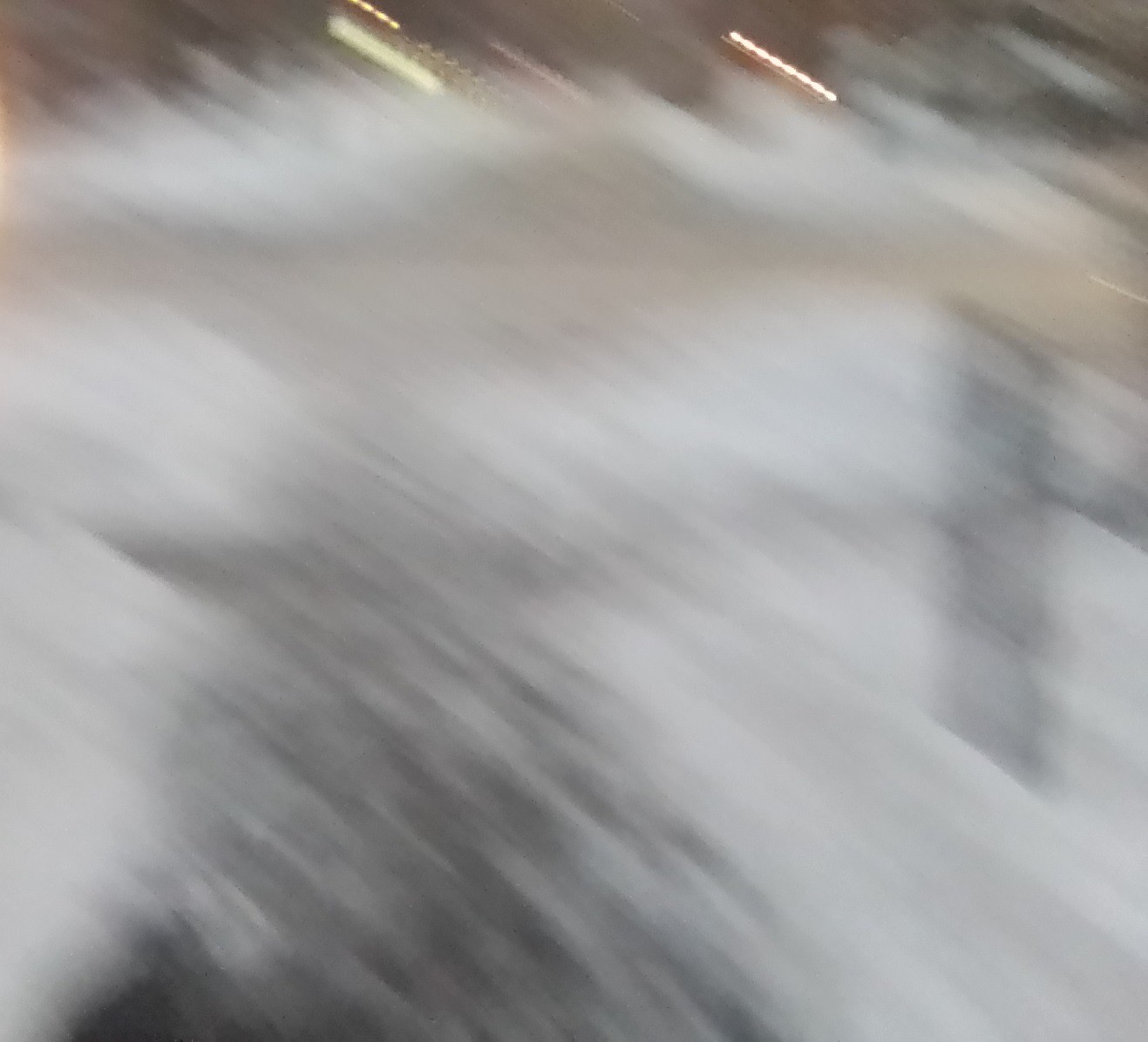The image portrays a winter scene with heavy snowfall blanketing both the foreground and background. Snow covers the ground extensively on the left and right, creating a thick, white layer. A partially cleared pathway or walkway, possibly shoveled out or cleared by some other means, divides the scene, leading diagonally from the top left to the bottom right of the image. The ground of this pathway appears to be made of stone or concrete.

The scene is noticeably blurred, adding an ethereal quality to the image, with lighting effects contributing to this sense of motion. Distant lights, likely streetlights or building lights, are visible in the sky at the top of the image, further enhancing the atmosphere. On the right side of the path, a series of red lights punctuates the scene, adding a contrasting color and drawing the eye. Snow-covered poles or posts are also visible, indicating some sort of structure or boundary within this wintry landscape.